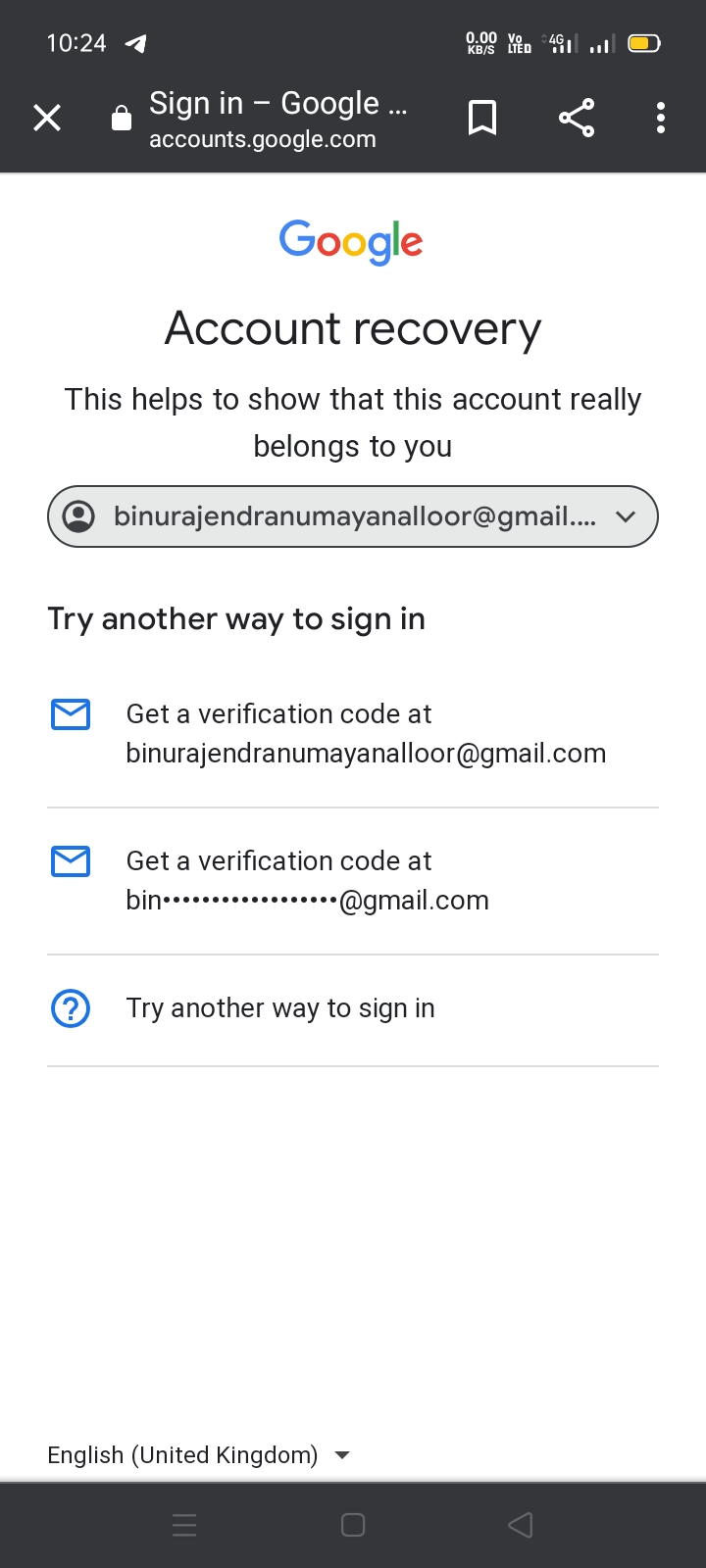In the image, an account recovery process for Google is underway. The top of the screen features the iconic Google logo in its signature rainbow colors. Just beneath the logo, the text reads "Account Recovery." A message below this states, "This helps to show that this account really belongs to you," emphasizing the security verification process.

Displayed prominently is a long Gmail account, partially obscured with asterisks in the middle to maintain privacy. The screen provides multiple options for verification, including "Get a verification code" sent to the listed Gmail, and the possibility to "Try another way to sign in."

At the bottom left of the screen, the language settings indicate "English (United Kingdom)," while a black bar at the bottom includes navigation symbols: three lines, a square, and a back button.

The top of the screen hosts a black status bar displaying the current time (10:24), battery life in orange, and icons for exiting, signing in through Google, bookmarking, and sharing. The overall background is plain white, with only the critical elements like verification options, the mail icons, and the Google logo adding splashes of color.